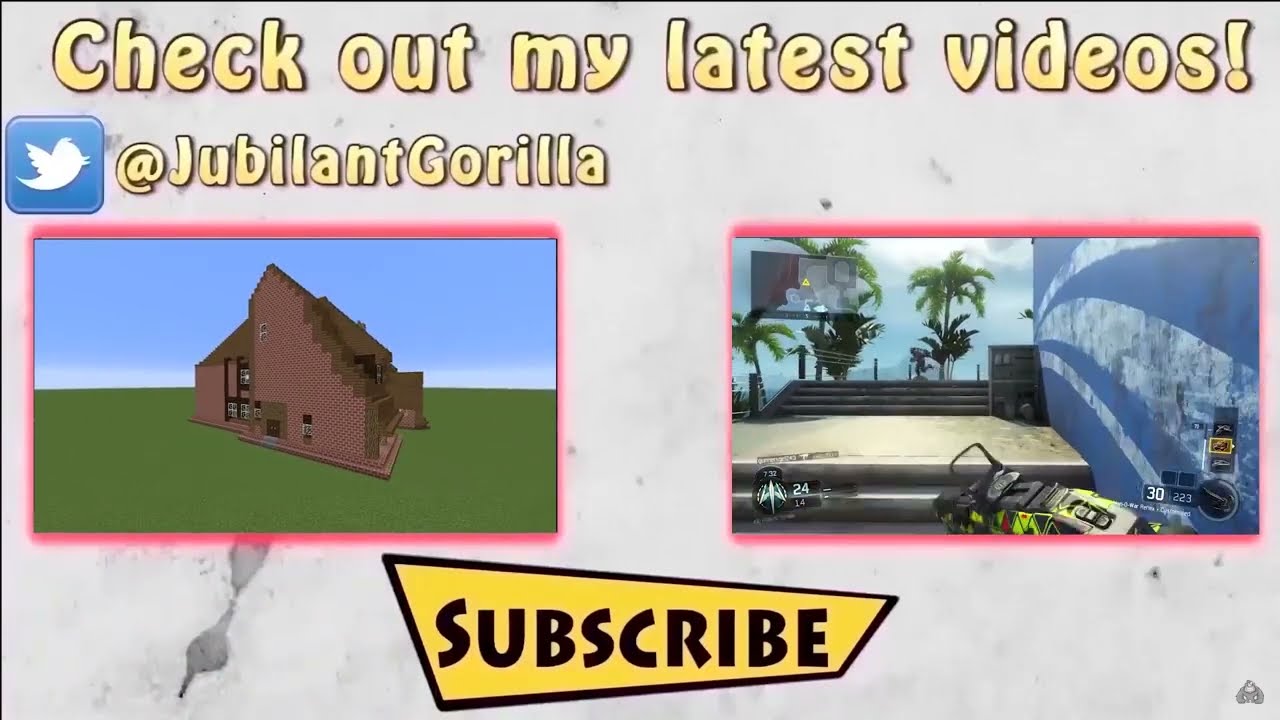This image is a screen capture from the popular video game Minecraft, likely taken from a YouTube video. The top of the image features a gray bar with light blue text reading "Make sure to subscribe for more." The word "subscribe" is prominently displayed in a red box with a right-pointing red arrow and a YouTube play button logo. In the upper right corner, there is a square with a red heart and another square that appears to have an umbrella icon.

The game interface at the bottom center shows the player's lives as blue hearts. Below this, there are several squares indicating various item quantities, such as 15, 20, 14, 40, 10, and 2. Just above these, a green bar with the number 7 displays the player's current level.

The in-game environment features a pathway that transitions from gray to brown to light brown and back to gray, running through a collection of structures built from concrete blocks. On the left side, steps fashioned from blocks lead up to a structure, whereas on the right side, gray blocks intermingle with wooden blocks in light and dark brown shades. In the middle slightly to the right, sloped hills with trees are visible, set against a white sky background. There is also some green on the ground, representing grass. The bottom right corner of the image shows the player's held item, adding to the detailed and immersive game scene.